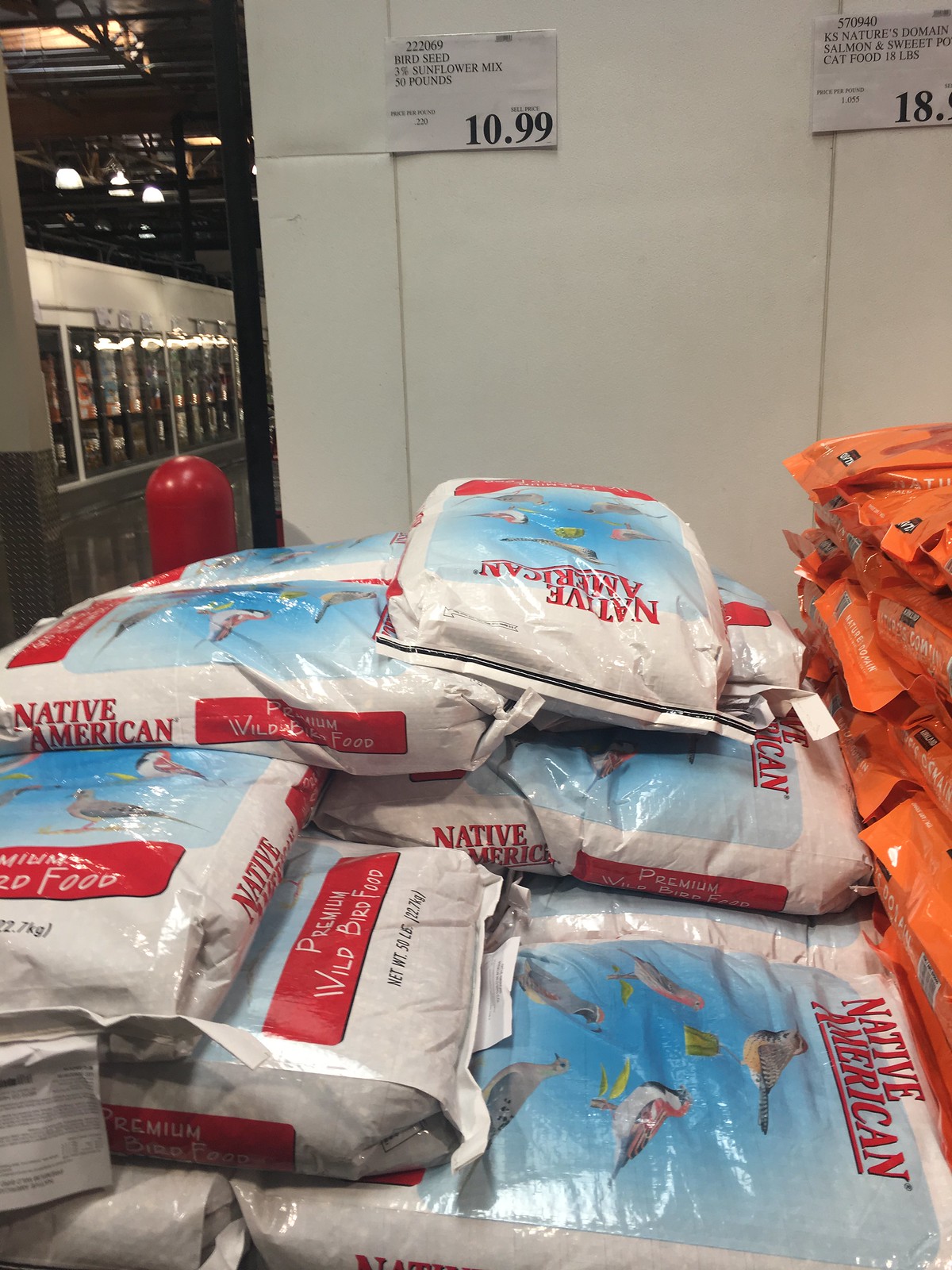In this image taken inside a store, there is a prominent display of a large bag of bird food labeled as Native American. The white bag is adorned with various illustrations of birds in a range of colors including red, white, and gray, all set against a striking turquoise background. The detailed design on the bag showcases different bird species and highlights the vibrant packaging. This sizable bag of bird food is priced at $10.99. Adjacent to it, there is another product with an orange bag priced at $18 and change, though the content and details of this product are obscured and not clearly visible. The scene is set against a white wall, and further into the image, there are metal cases containing assorted foods.